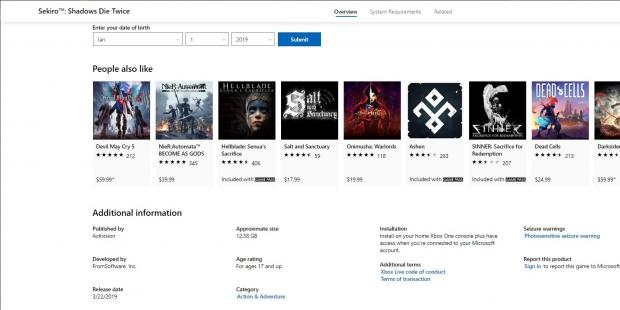The image is a screenshot of a somewhat blurry website displaying information about the game "Sekiro: Shadows Die Twice." In the top left corner, there is a prompt to enter your date of birth (month, day, and year) to proceed. Below this prompt, various cover images and icons of games that users might also like are featured, including titles like "Devil May Cry" and "Salt and Sanctuary." 

A section labeled "Additional Information" provides details such as the publisher, developer, release date, and categorizes the game under "Action and Adventure." The website showcases a total of nine images, but only part of the ninth image and its text are visible. Prices are listed beneath each image, giving viewers an idea of the cost of each game.